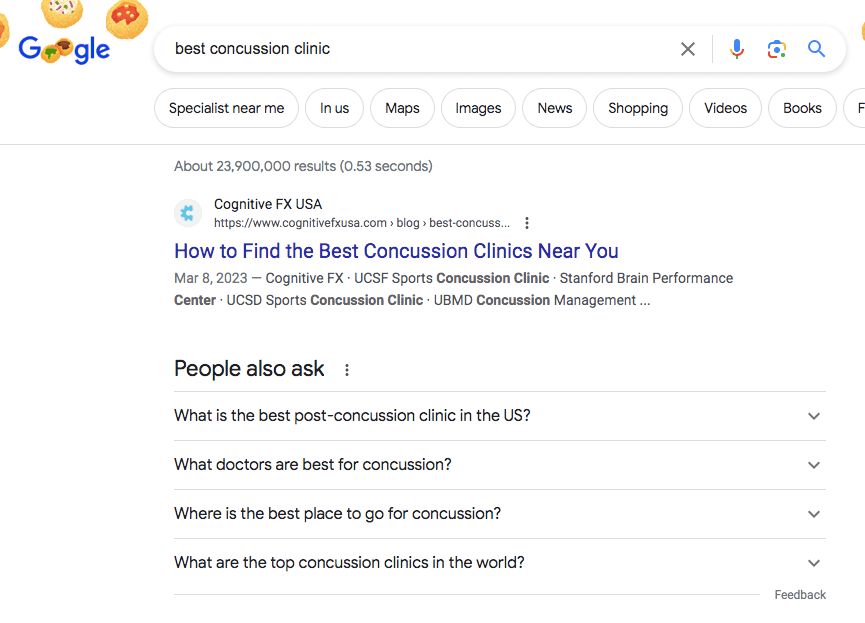The image features a clean, white background with a Google search interface prominently displayed. On the left side of the image, there are small cookies decorated with various toppings. The Google logo, in its characteristic blue, is positioned above two centrally-placed cookies, one topped with green sprinkles and the other with brown. Surrounding these are three additional cookies.

Below the cookies is a search bar containing the text "best concussion clinic." At the end of the search bar are an "X" icon and a microphone icon. Adjacent to the search bar is a small blue square with red, blue, and yellow elements, centered with a blue dot, and a magnifying glass icon for initiating searches.

Below the search bar are several navigation buttons: "All," "Specialists near me," "In US," "Maps," "Images," "News," "Shopping," "Videos," and "Books." To the right of these is an "F" enclosed in a circle, followed by a light blue line separating the navigation section from the search results.

The search results indicate approximately 23,900,000 results found in 0.53 seconds. The first result is from Cognitive FX, USA, under the heading "How to find the best concussion clinics near you." Below this search result is a "People also ask" section featuring expandable questions: 
- "What is the best post concussion clinic in the US?" 
- "What doctors are best for concussion?" 
- "Where is the best place to go for concussion?" 
- "What are the top concussion clinics in the world?" 

Each of these questions has a corresponding down arrow for further expansion. At the bottom of this section is a "Feedback" link.